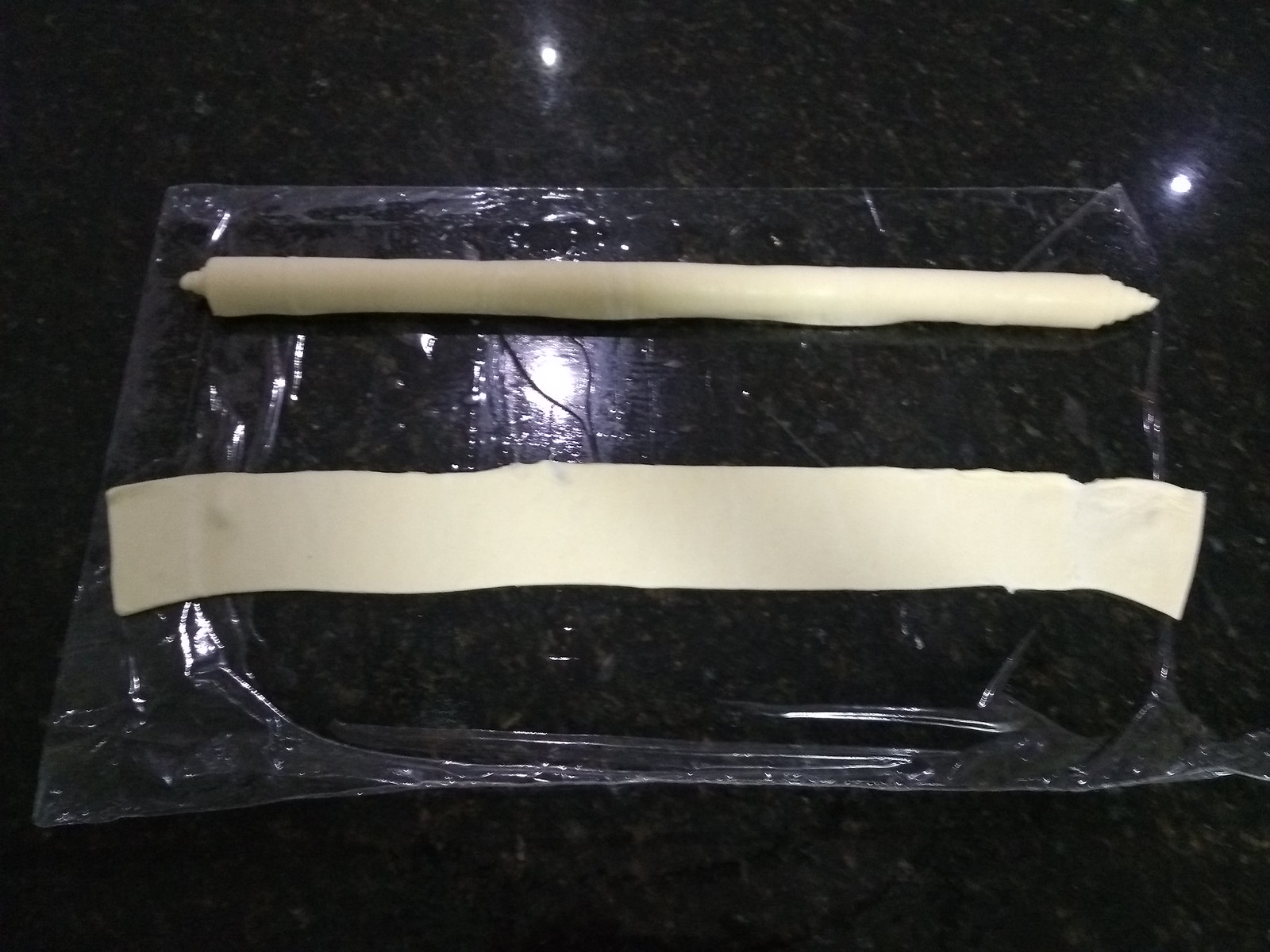An overhead image captures a black, faux-marble countertop, distinguished by its spotty black and gray appearance and three small white light reflections—two above and one amid the items on the surface. Positioned centrally is a clear plastic sheet, upon which lie two strips of tan-colored dough-like material. The top strip is rolled up into a cylinder with tapered ends, while the bottom strip remains flat, long, and slightly curving like a rectangle. The overall scene showcases the intricate play of light and materials on an elegantly textured black marble-like background.